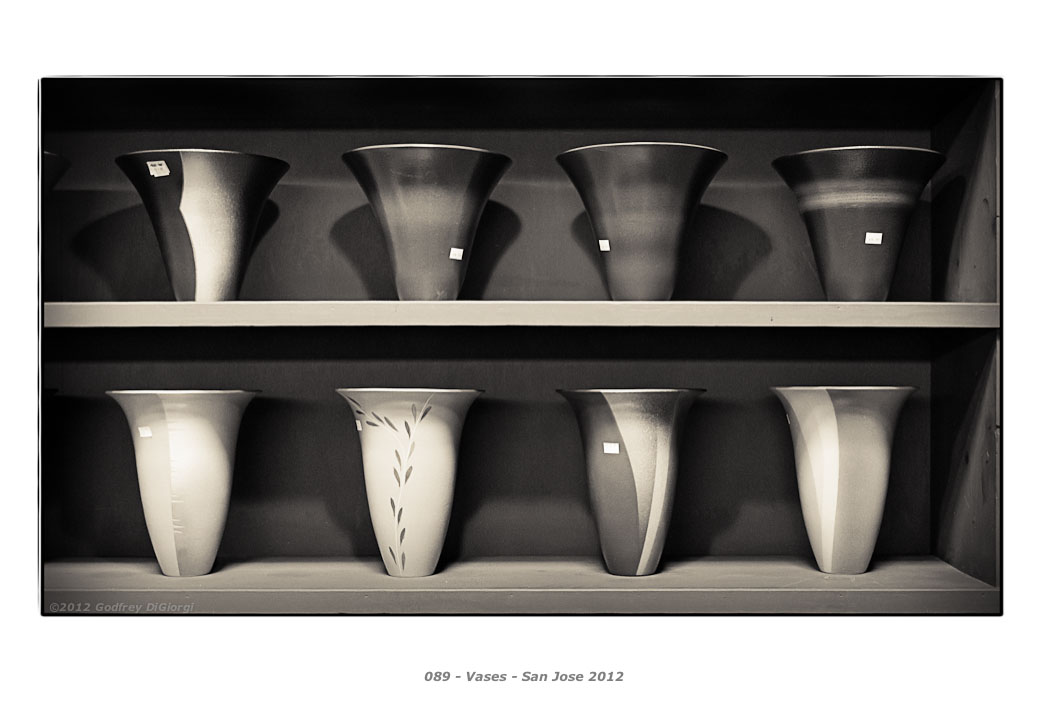This is a detailed black-and-white photograph depicting eight vases arranged on two shelves, with four vases on the top shelf and four on the bottom shelf. The shelves themselves have a dark gray background, with the ceiling of the upper shelf appearing black and the base of the lower shelf a light gray. 

The vases on the top shelf have a fluted shape, starting thin at the bottom and widening out at the top. The top left vase features a curved stripe pattern, although the designs on the other vases are primarily subtle swirls, with little variation in shades due to the grayscale nature of the photograph.

On the bottom shelf, the vases have an inverse bell shape, narrower at the base and more rounded in the middle with a wide lip around the top. One vase on this shelf, the second from the left, has a simple pattern resembling a stalk with small leaves. The third and fourth vases exhibit abstract stripes of varying sizes and orientations. Each vase has a small white tag attached to it.

Below the photograph, there is a block of grey text labeled "089-Vases-San Jose 2012." Additionally, a low-opacity watermark reading "2012 Godfrey DiGiorgi" is located in the photograph's lower left corner, acknowledging the artist.